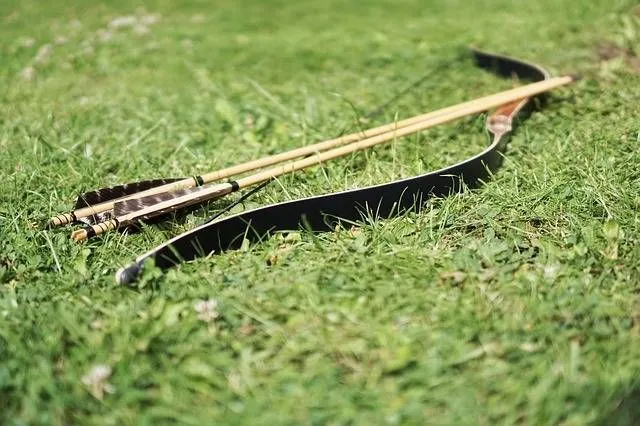This horizontal rectangular image captures an elaborate black longbow and two arrows carefully placed on top of it in a grassy area. The bow and arrow set seems to have been cautiously set down after use. The two arrows, made of light tan wood, rest diagonally across the bow from corner to corner. They feature brown and white striped feathers at their notched ends, designed for easy attachment to the bowstring. The grass, appearing manicured and about 2 to 3 inches high, provides a vibrant green backdrop. The bowstring stretches taut from the top to the bottom of the bow, accentuating its readiness for action. Despite some blurriness in the image, the precision of the arrows' feathers and the meticulous placement suggest a scene of careful preparation or momentary pause in archery activity.